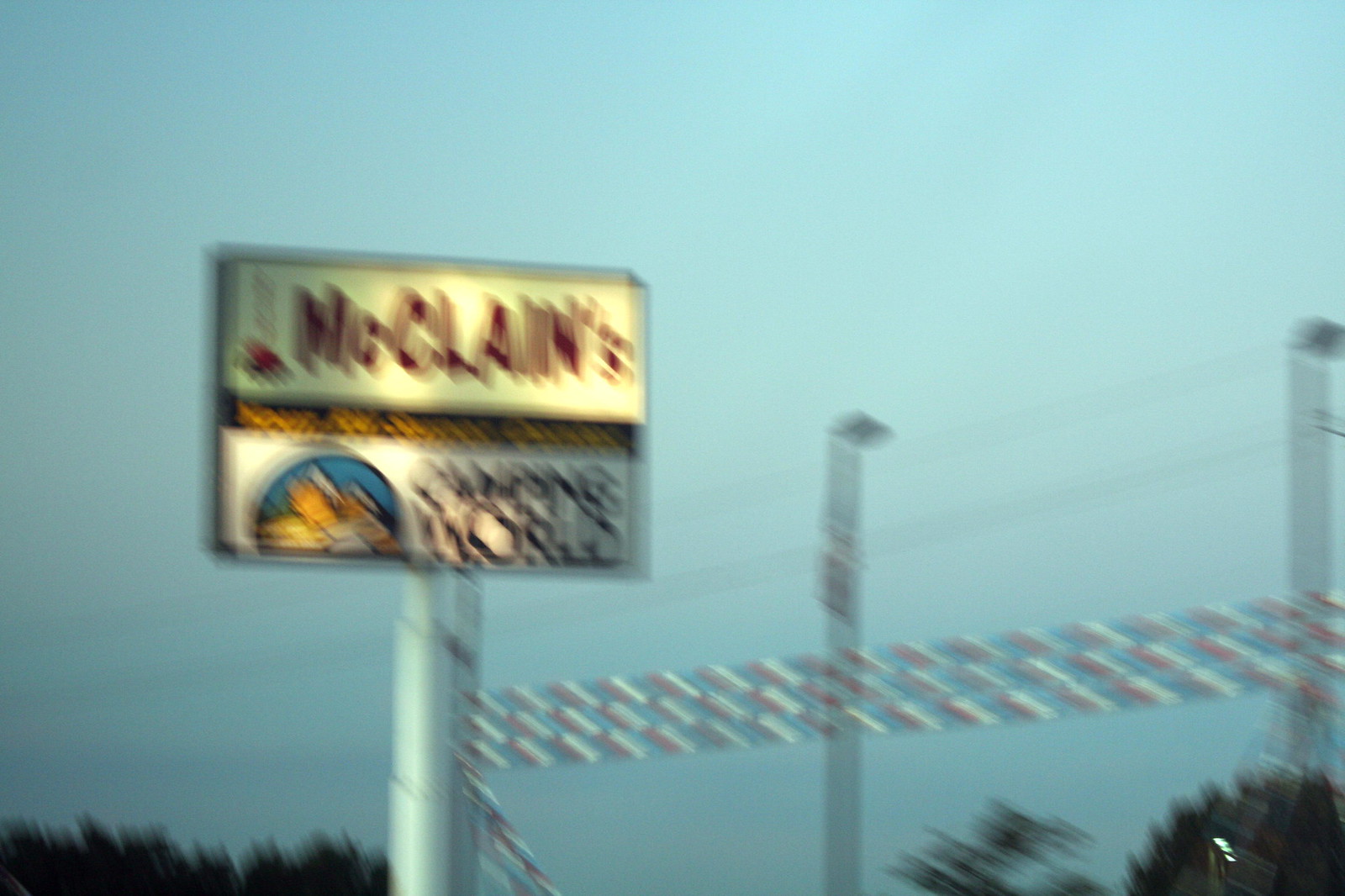The image shows a very blurry sign for a business situated against a backdrop of a blue sky with a few scattered white clouds. The sign features a yellow background at the top with red text reading "McLean's." Below that, there's a small gold and black border, followed by a white background displaying a logo with the text "Camping World." The sign is mounted on a tall, round, white pole that extends downward out of the frame. From the side of the pole, several rows of plastic ribbons, likely colored and designed to wave in the breeze, extend off-image. In the background, there are light or power poles with lines stretching between them, as well as the tops of some trees. The lighting in the image is low, suggesting it was taken either at sunrise or sunset. The sky is predominantly blue with minimal cloud cover.